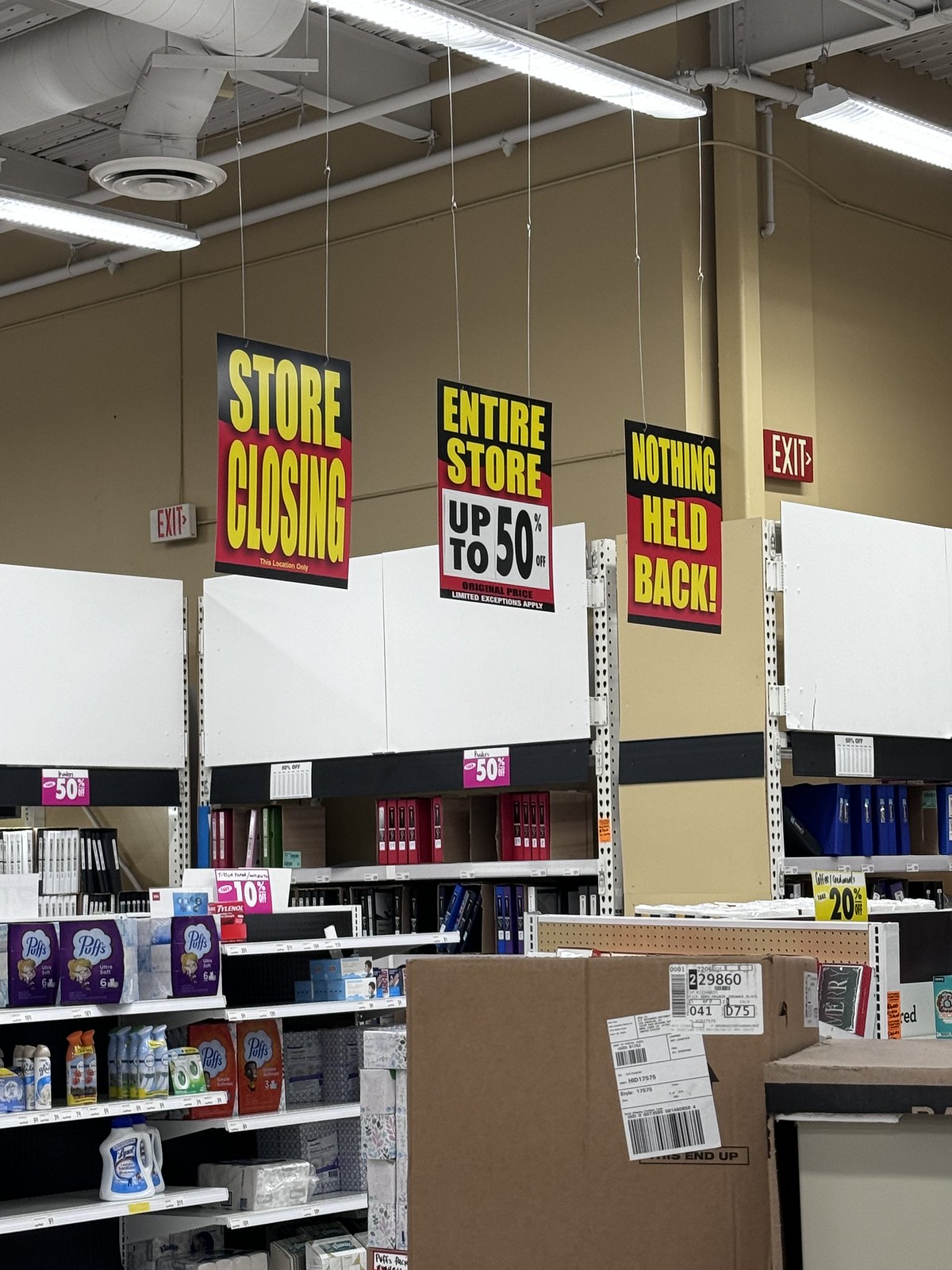This photograph depicts the interior of a large retail store with towering 25 to 30-foot high ceilings supported by visible gray pipes and conduits. Three prominent signs hang from the ceiling by wires above the shelves: the leftmost sign, half black and half red, proclaims "STORE CLOSING" in yellow text; the central sign, similarly colored, reads "ENTIRE STORE" in yellow, followed by a white rectangle with black text stating "UP TO 50% OFF;" and the rightmost sign, also black and red, declares "NOTHING HELD BACK!" in yellow. Below these signs, numerous shelves display a variety of discounted items, including toilet paper, cleaning products like pump sprays and aerosol sprays, and what appears to be napkins and binders. The overall impression is of a store undergoing a closing sale, offering various discounts. Additional details include a light brown upper wall, a series of fluorescent light fixtures suspended from the ceiling, a red exit sign, and white shelving dividers, all contributing to the visually cluttered but clearly marked environment of a store in its final days of operation.